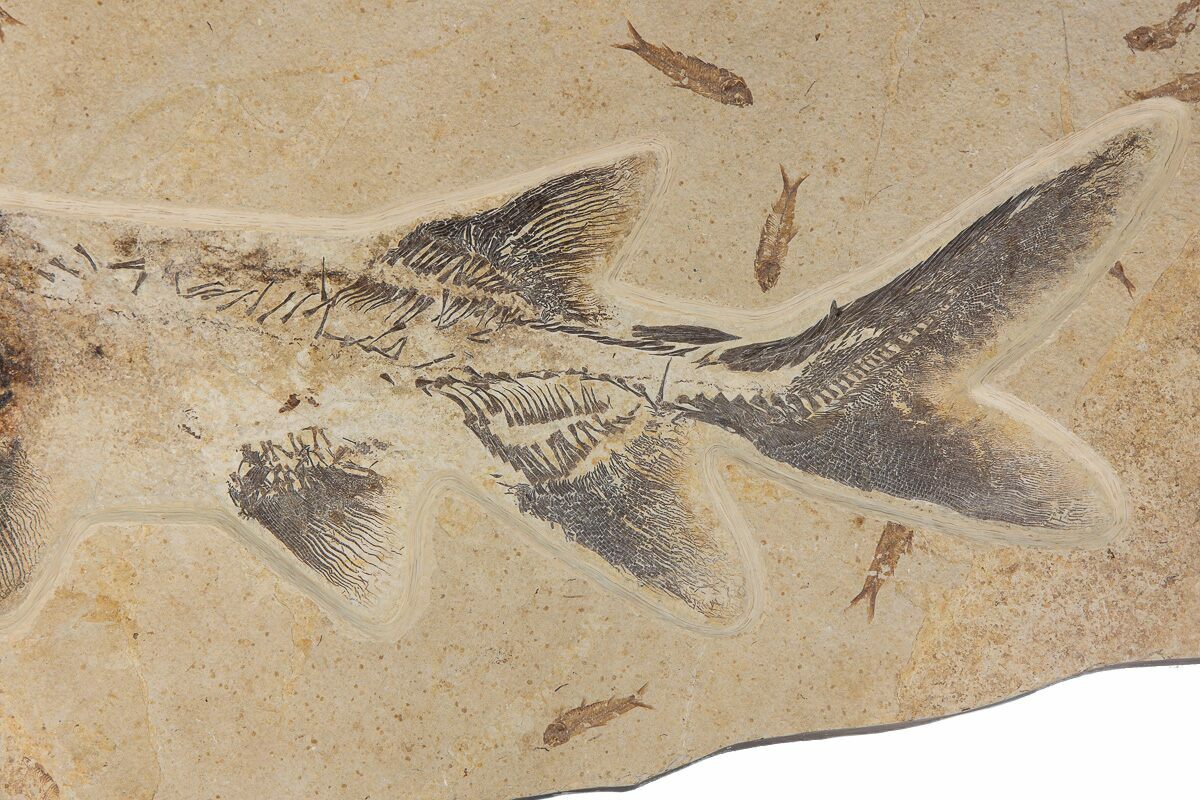The image depicts a detailed fossil embedded in a tan and beige sandstone, possibly found on a beach. Central to the fossil is a large fish, its skeletal remains displaying distinct scales and bones, with visible fins on both sides and a larger fin on its back. Part of the fish appears partially buried in sediment, giving it a darker grayish-charcoal hue. Surrounding this main specimen are seven smaller fish, each identifiable by their simple fin structures. The scene captures a dynamic underwater moment, possibly resembling a cave painting but clearly showcasing the movement of these ancient aquatic creatures.